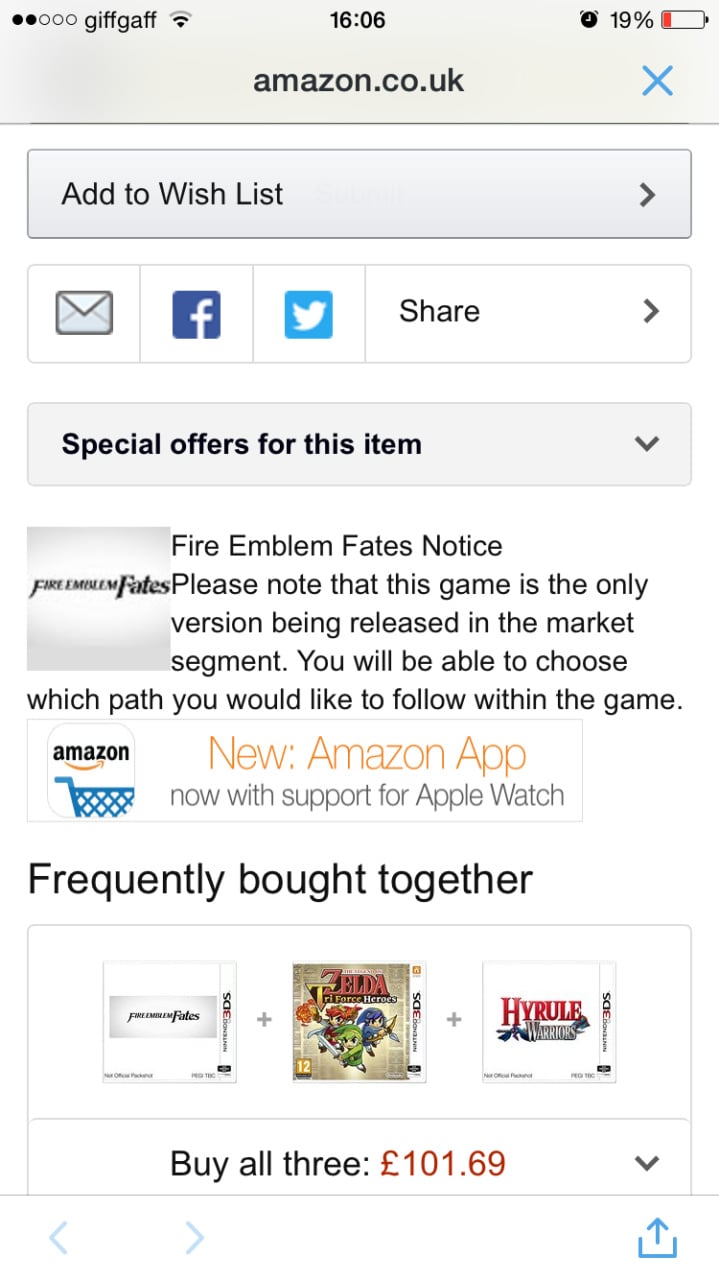A user has clicked on a link leading to the Amazon UK website, specifically at the address "amazon.co.uk." It appears they might have clicked on an advertisement or some kind of link embedded within another site, as the Amazon page is opened externally. Upon arrival, the user finds themselves on a product page, though the product image is not immediately visible. As they scroll down, they see various buttons, including an "Add to Wishlist" button, multiple share buttons for social media, and special offers related to the item.

The product in question is "Fire Emblem Fates," which comes with a notice indicating that this particular version is the only one being released in that market segment. The information reveals that players can choose their path within the game. Additionally, there is a "Frequently Bought Together" section showcasing "Fire Emblem Fates" alongside two "Zelda" games, indicating some similarities or a shared audience between the franchises.

The page features a predominantly white background with extensive black text, making the details clear and readable. The user notes the connection to Zelda games, suggesting that "Fire Emblem Fates" shares thematic or gameplay elements with the Zelda series. Further scrolling is necessary to see more details or proceed with the checkout process.